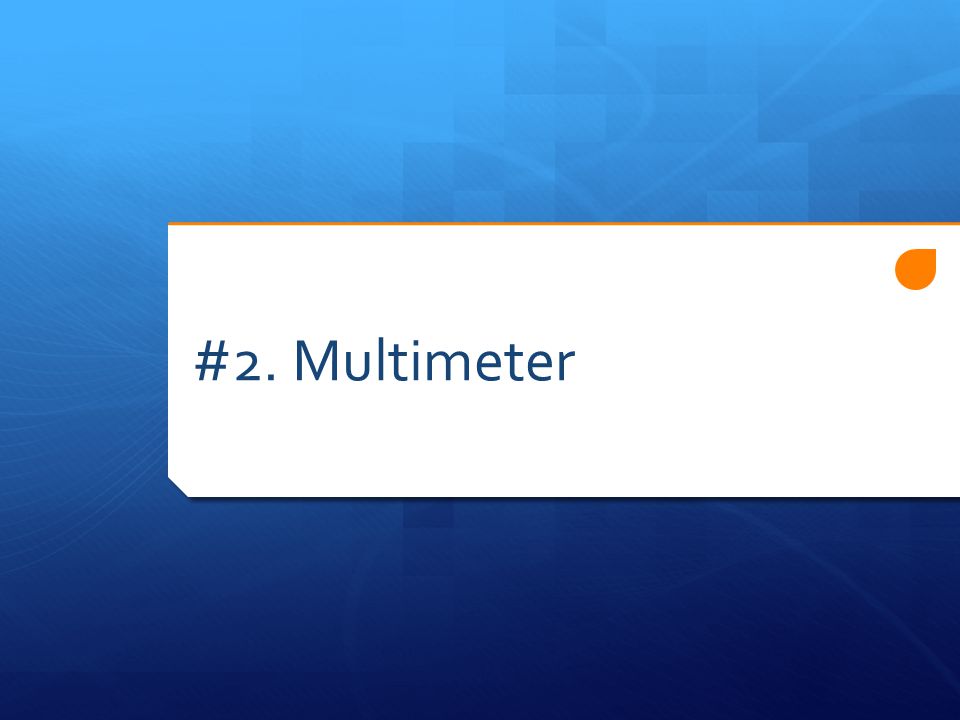The image appears to be a slide from a PowerPoint presentation, formatted in landscape orientation. The background features a gradient that transitions from light blue at the top to deep navy blue at the bottom. Superimposed on this gradient are subtle elements like squares and swirls, adding a minimalist touch. 

Dominating the center is a white rectangular tab that extends from the right, covering about a third of the image's height and three-quarters of its width. The rectangle's bottom left corner is clipped at an angle, giving it a distinctive shape. At the top of this white rectangle is a narrow goldish-orange line, and to its top right corner is an orange teardrop icon.

Centered within the white rectangle, in dark blue font, is the text "#2. Multimeter." The overall style of the slide leans towards a clean and simple color infographic, prioritizing clear visual hierarchy and minimal distraction.